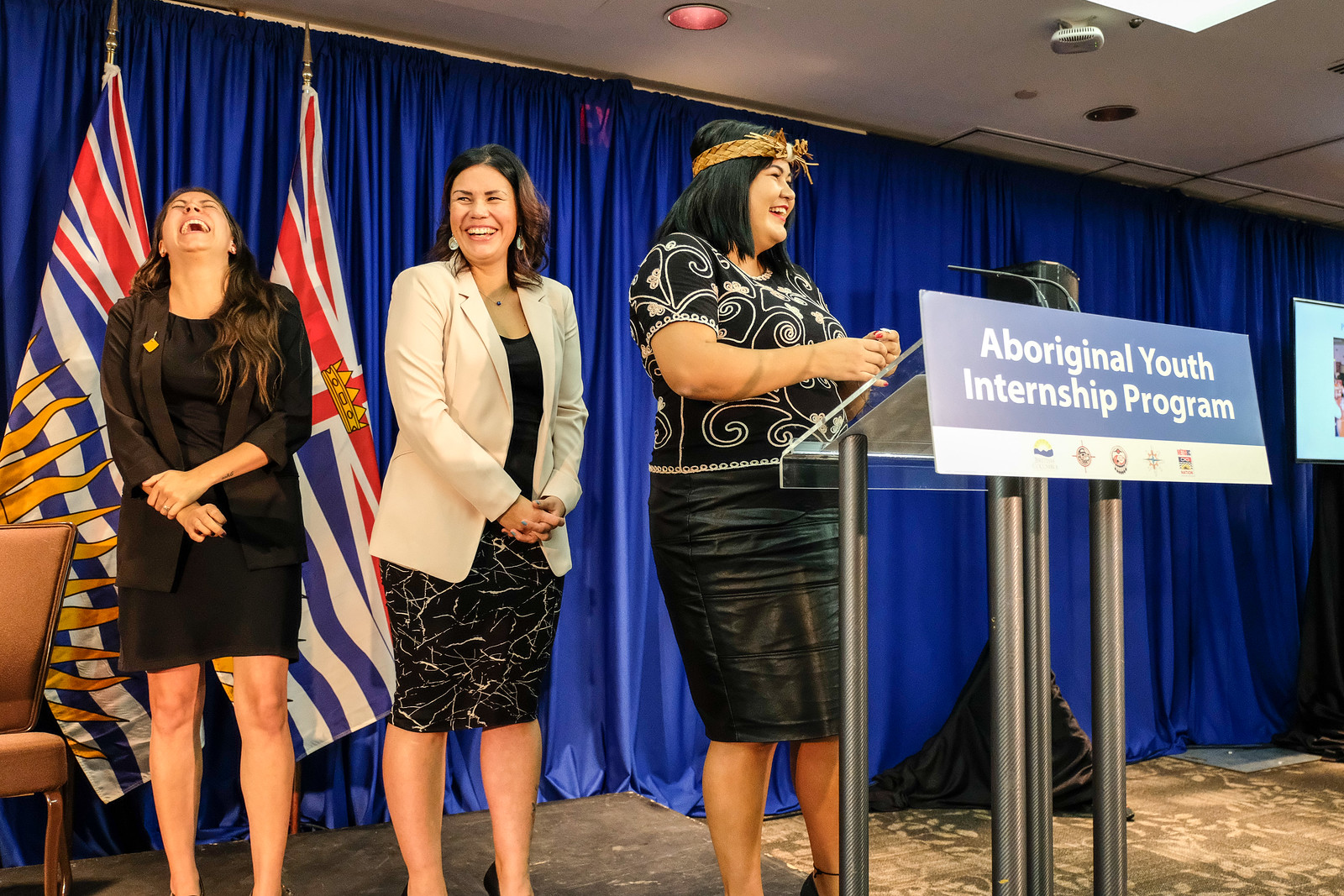In this vibrant color photograph, three young women of Aboriginal descent stand on a stage, clearly enjoying a moment of shared laughter during a presentation for the Aboriginal Youth Internship Program. The scene is set against a backdrop of a blue curtain and two flags, with one flag featuring the Union Jack and a pattern of blue and white lines. A sleek podium bearing a sign with the program's name and various sponsor logos stands to the right.

The young woman at the center of the image exudes confidence and joy. She wears a striking black and white swirl top paired with a black leather skirt and a festive lei on her head. Her smile is radiant as she glances off to the right. To her left, another young woman in a white jacket and black and white skirt also beams, clearly amused by the moment. The third woman, donned in an all-black ensemble, is equally engaged, her head thrown back in hearty laughter. Their business-professional attire underscores the importance of the event, while their expressions and body language communicate a sense of camaraderie and excitement. The overall atmosphere is lively and positive, capturing a memorable and uplifting slice of this significant program.